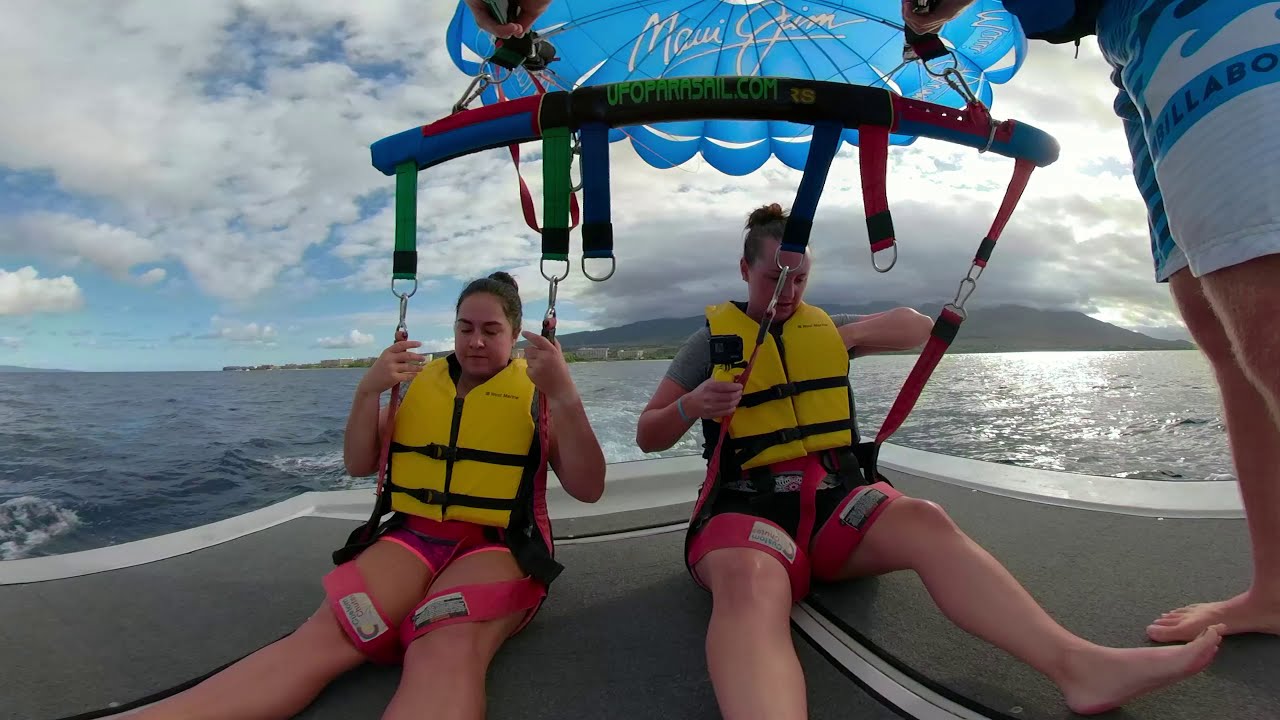The image captures two people sitting at the back of a boat, preparing for a parasailing adventure. Both individuals are clad in swimsuits and identical yellow life vests secured with two buckles and belts on the front. The person on the right wears a short-sleeved green shirt and has a black GoPro camera attached to their life vest, while the person on the left is donned in a one-piece pink swimsuit with longer leggings featuring black stripes on the sides. The harness system, composed of pink and black straps around their legs and waist, is connected to a large D-ring and a prominent handle inscribed with "ufoparasail.com". The background reveals a cloudy sky with hints of blue, a distant hill, and ocean water filled with the boat's wake. A man, visible only by his legs and shorts, stands to their right, seemingly instructing them. The two appear slightly apprehensive as they face the upcoming excitement of their parasailing experience. Behind them, a blue sail readies for their lift-off.